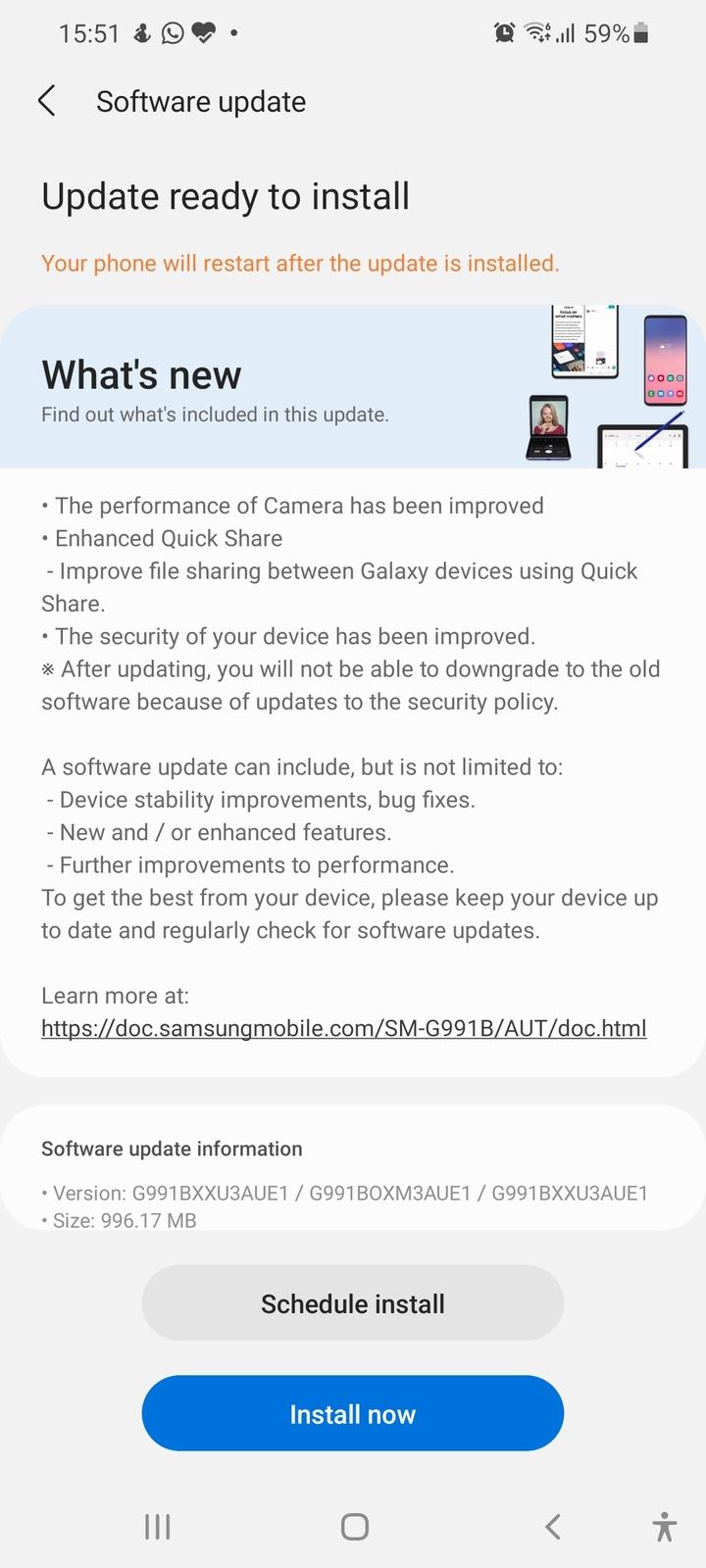A detailed view of a smartphone screen displaying a software update notification.

- **Time and Status Icons**: The phone indicates the time as 15:51 (3:51 PM), displayed on a gray background. On the upper right, the status icons include an alarm clock, Wi-Fi signal, signal strength bars, and a battery indicator showing 59% charge.

- **Update Notification**: At the top of the screen, in bold black text, it says "Software update" alongside a less-than symbol. Below, in black text, it states, "Update is ready to install."

- **Installation Reminder**: Highlighted in orange text, it reads, "Your phone will restart after the upgrade is installed."

- **What’s New Section**: A rounded rectangle box with "What's new" in bold is present. The text "Find out what's included in this update" appears in regular font. Displayed are various icons and images depicting a woman on a flip phone, an iPad displaying news, a smartphone home screen, and a tablet with numerical data and a pen.

- **Update Details with Bullet Points**:
  - The performance of camera has been improved.
  - Enhanced quick share.
    - Improved file sharing between Galaxy devices using quick share.
  - The security of your device has been improved.
  - Note: After updating, you will not be able to downgrade to the old software due to security updates.

- **Additional Information**: 
  - "A software update can include but is not limited to":
    - Device stability improvements.
    - Bug fixes.
    - New and/or enhanced features.
    - Further improvements to performance.

- **Recommendation**: "To get the best from your device, please keep your device up to date and regularly check for software updates." A URL link to learn more is provided: https://doc.samsungmobile.com/.sm-g991b-aut-doc.html.

- **Software Update Information**: Encased in an oval-shaped white box:
  - Version: G991BXXU3AUE1 / G991BOXM3AUE1 / G991BXXU3AUE1.
  - Size: 996.17 megabytes.

- **Installation Buttons**:
  - "Schedule install" in black text with a gray background.
  - "Install now" in white text with a blue oval background.

- **Screen Bottom Icons**: At the bottom, icons include three vertical lines, a rounded rectangle, a less-than symbol, and a small figure icon.

In the upper portion of the screen, a small black dot and a speech bubble with a phone inside and a heart with a zigzag line are also noted.